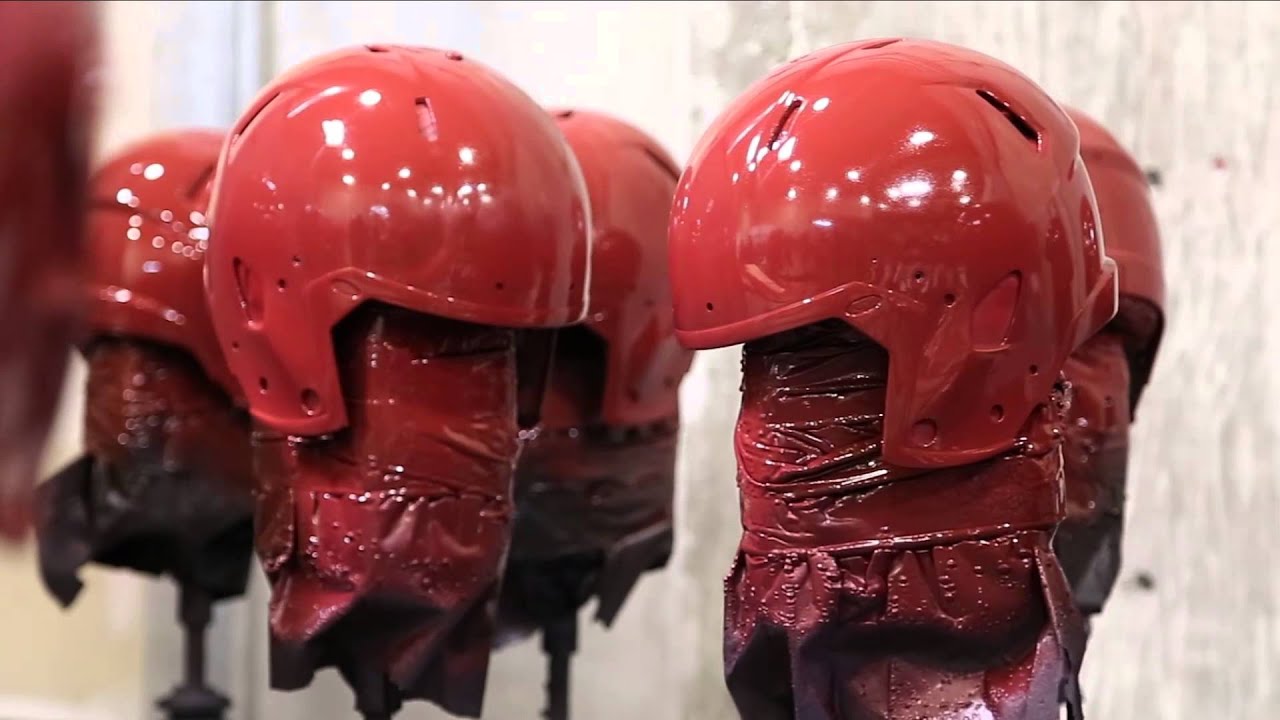The image depicts five red helmets prominently displayed on what appear to be red, padded poles, possibly spray-painted, with a black base at the bottom. Each helmet covers the head, leaving the front open, and extends to protect the ears. There are rectangular ventilation holes at the top of each helmet to allow air circulation. Two helmets are clearly visible in the foreground while three more are positioned in the back. All helmets appear wet and slick, indicating they were recently painted. The background is a bit blurry, but a white concrete wall and indistinct dark shapes can be vaguely made out, suggesting a spacious area possibly resembling a multi-story building.